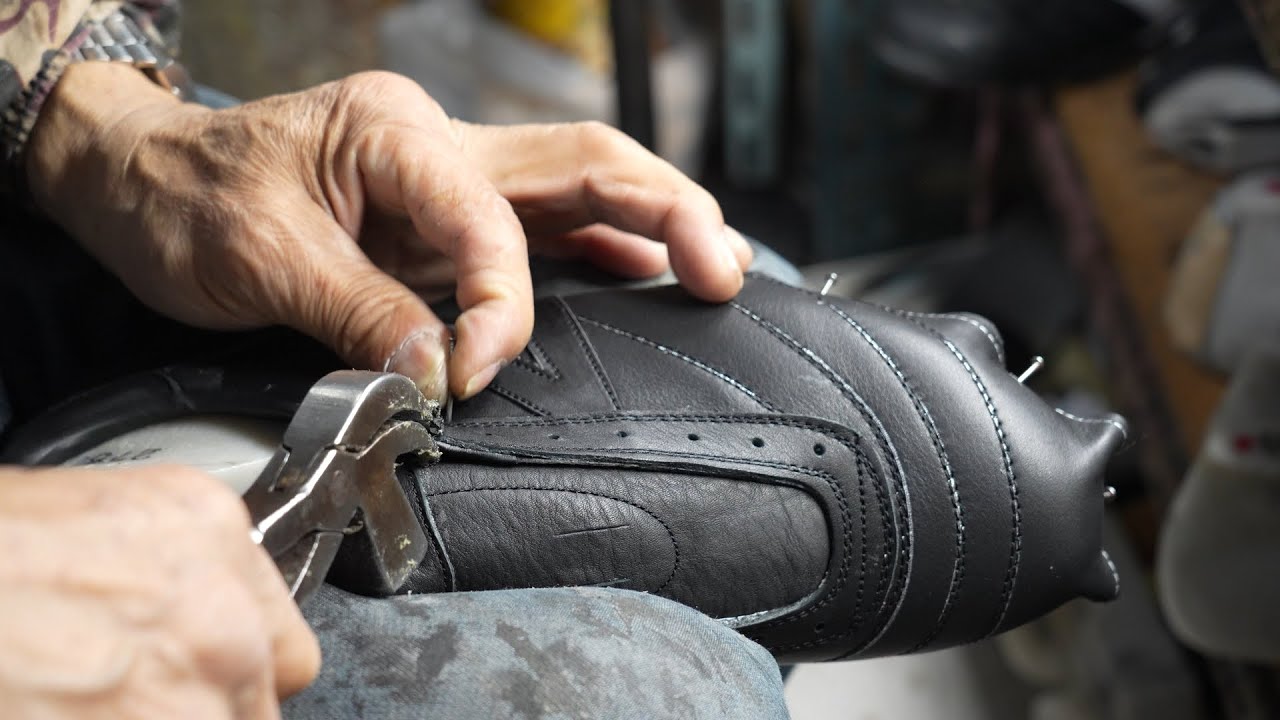In this highly detailed, close-up image, an older individual's hands—pale, weathered, and calloused—are meticulously working on a black leather sneaker. The person holds a pair of metal pliers in their right hand, using it to punch holes for the shoelaces in the leather, which is partially wrapped around the shoe’s sole and secured with small nails. The background of the image features various tools and benches adorned with folded materials, hinting at a well-used workspace of a skilled cobbler. A man's watch is subtly visible in the top left corner, adding a touch of context to the craftsman’s identity, suggesting experience and dedication to the craft. The horizontal orientation of the photograph, despite some imperfections in lighting and texture, captures the essence of traditional shoemaking.